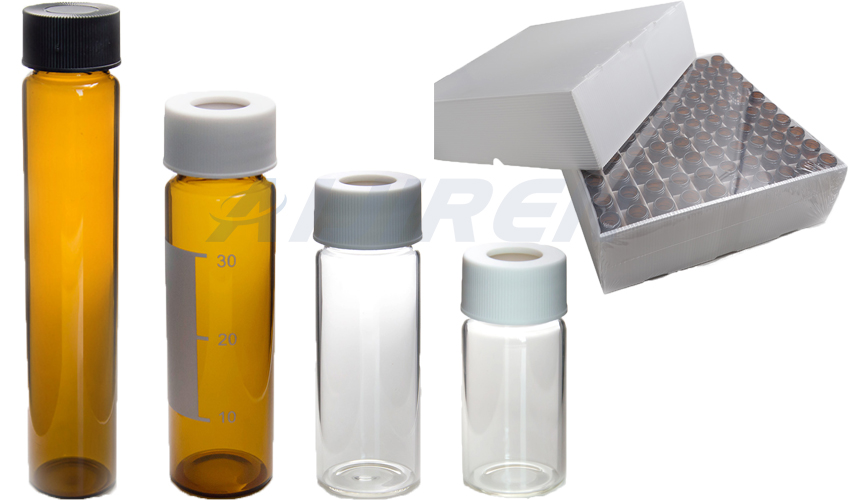This image depicts an array of four vials positioned in a row, each descending in height from left to right. The leftmost vial is the tallest and features a black screw top with rich amber-colored glass. The second vial, slightly shorter, also has an amber tint and is topped with a white cap, bearing measurement markings for 10, 20, and 30 milliliters. The third vial is clear and equipped with a white cap, slightly smaller than the second. The rightmost vial is the shortest, clear in color, and also sports a white cap. Adjacent to these vials is an open, dull-gray box with a lifted top, suggesting a storage or shipment solution, containing compartments for housing additional vials. A partially visible name or logo is stamped over the image.